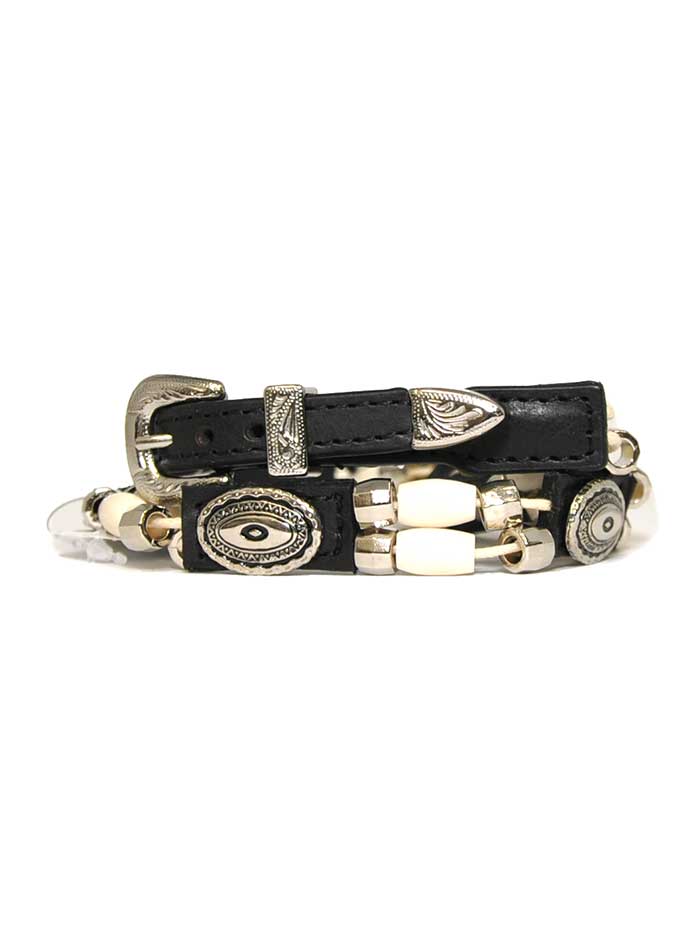This is a professional close-up photo of a black leather belt coiled up against a stark white background. The belt features intricate silver and chrome accents, giving it a decorative and almost Southwestern or Native American-inspired aesthetic. The buckle, prominently displayed on top, is adorned with silver etchings. The belt itself is sectioned with oval-shaped silver conchos, each intricately tooled. Between each leather section, there are beaded cords featuring silver and white beads, with smaller silver beads at the ends and a larger white bead in the middle of the cord. The detailed craftsmanship and beading make the belt look almost like a piece of jewelry, but the presence of the buckle and belt holes confirms its identity as a belt.